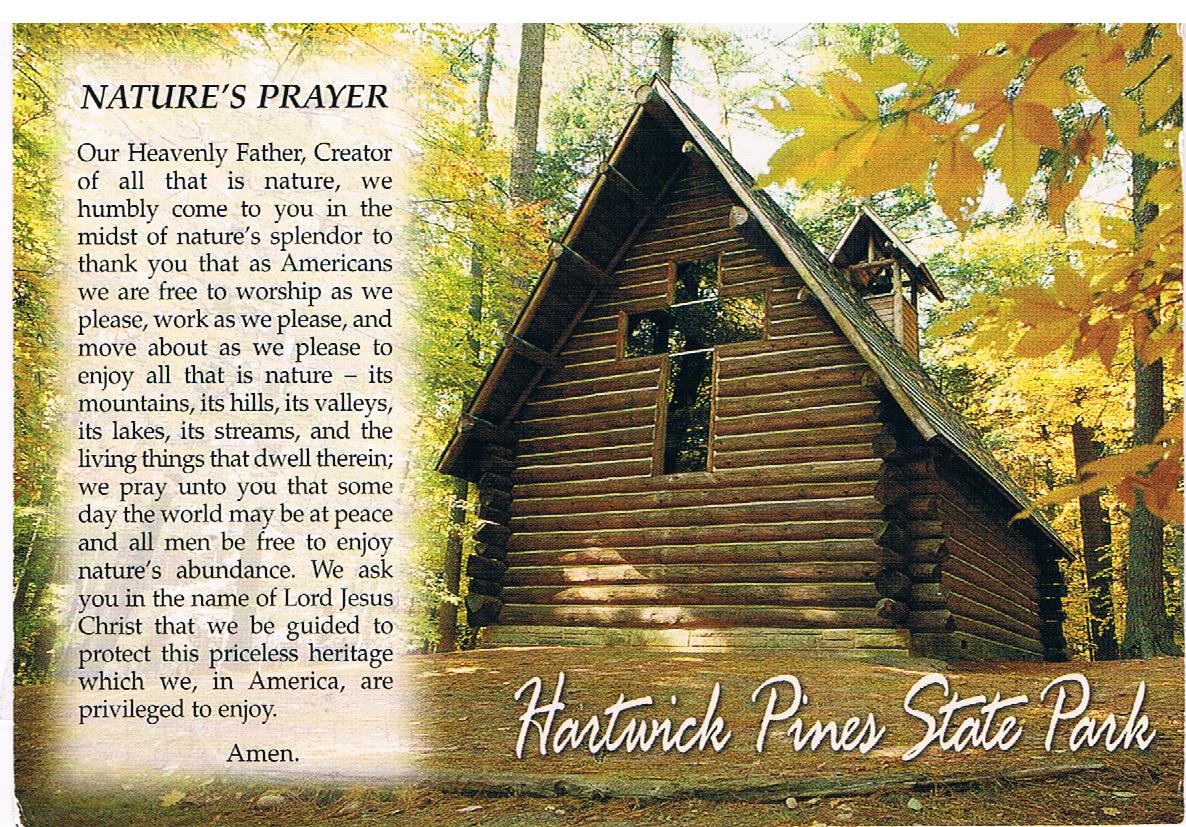The image depicts a log cabin church with a large cross-shaped window on its nearest wall, nestled deep within a forest adorned with vibrant autumn foliage of golden, orange, and brown leaves. A small bell tower or steeple is positioned at the far end of the cabin. The scene is set under a bright, sunny sky. In the foreground, there is a visually pronounced clearing with a large branch lying on the ground. On the left side, a feathered white text box contains the invocation, "Nature's Prayer," written in large black font with a white glow. Below, it continues with a heartfelt plea to the Heavenly Father, expressing gratitude for the freedoms Americans enjoy and a wish for global peace and preservation of nature's bounty. On the bottom right corner of the image, white cursive text proclaims the location as Hartwick Pine State Park.